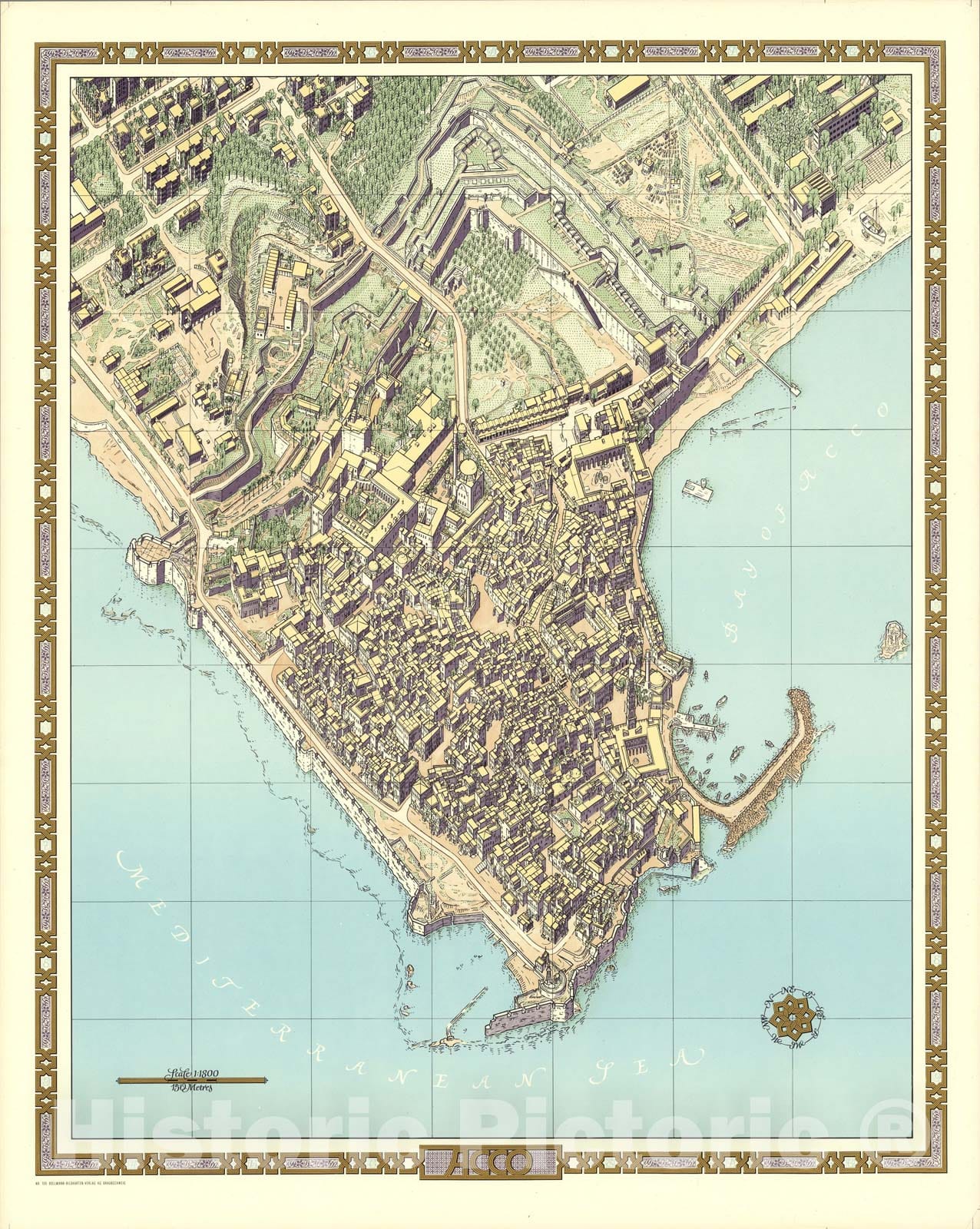This is an image of a historical map depicting a peninsula surrounded by a blue sea. The map itself appears aged, with faded colors. It features an ornate golden and gray border with a design incorporating rectangular patterns. Dominating the peninsula is a densely populated or developed area, mostly illustrated in light brown. As you move inland towards the base, the density of development decreases, showing more green rural areas. In the bottom left corner, there is a brown or golden legend, and a compass is situated at the bottom right. The top left section of the peninsula also retains some developed areas. The map’s outer edges have a beige-pink hue, complemented by a detailed border in brown, tan, and blue, and a final white border enclosing the map. The inscription "historic pictoric" with a circled 'C' is noted at the bottom, though details about the exact location remain unclear.